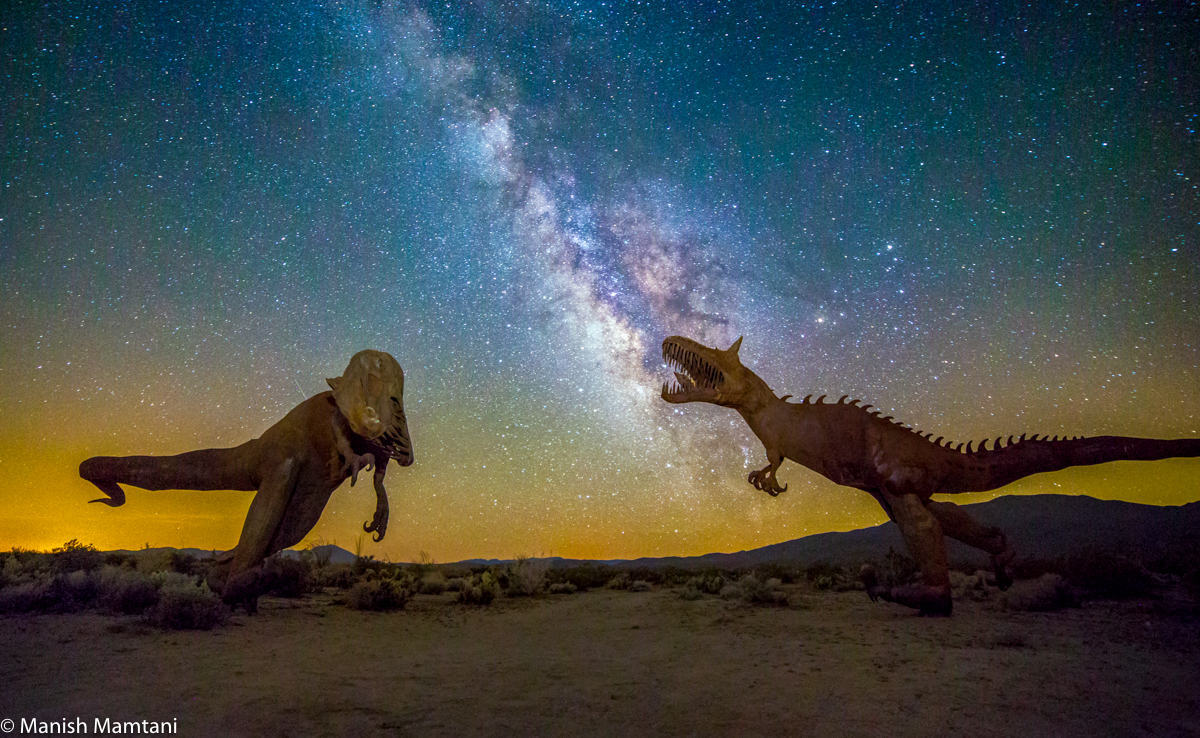In a surreal desert landscape under a vibrant night sky painted with swirling hues of cyan, purple, orange, and yellow, two dinosaur-like creatures face one another. Both creatures have thick legs with large feet, short arms with thin fingers, and elongated, sparse teeth. Spiky protrusions, resembling horns, extend from their spines, and each has two long ears that extend vertically from their heads. The creature on the right, light brown in color, has a large tail and features reminiscent of a T-Rex, with its menacing open mouth displaying long teeth. The creature on the left has a smaller head, turned at an angle, with an open mouth and a long tail. It stands awkwardly on its front legs, giving it a distorted appearance. The scene is made even more otherworldly by the short, varying shades of green foliage scattered on the ground. The digital artistry marks the bottom left corner with a copyright attribution to Manish Mamontani, completing the mesmerizing nocturnal tableau.